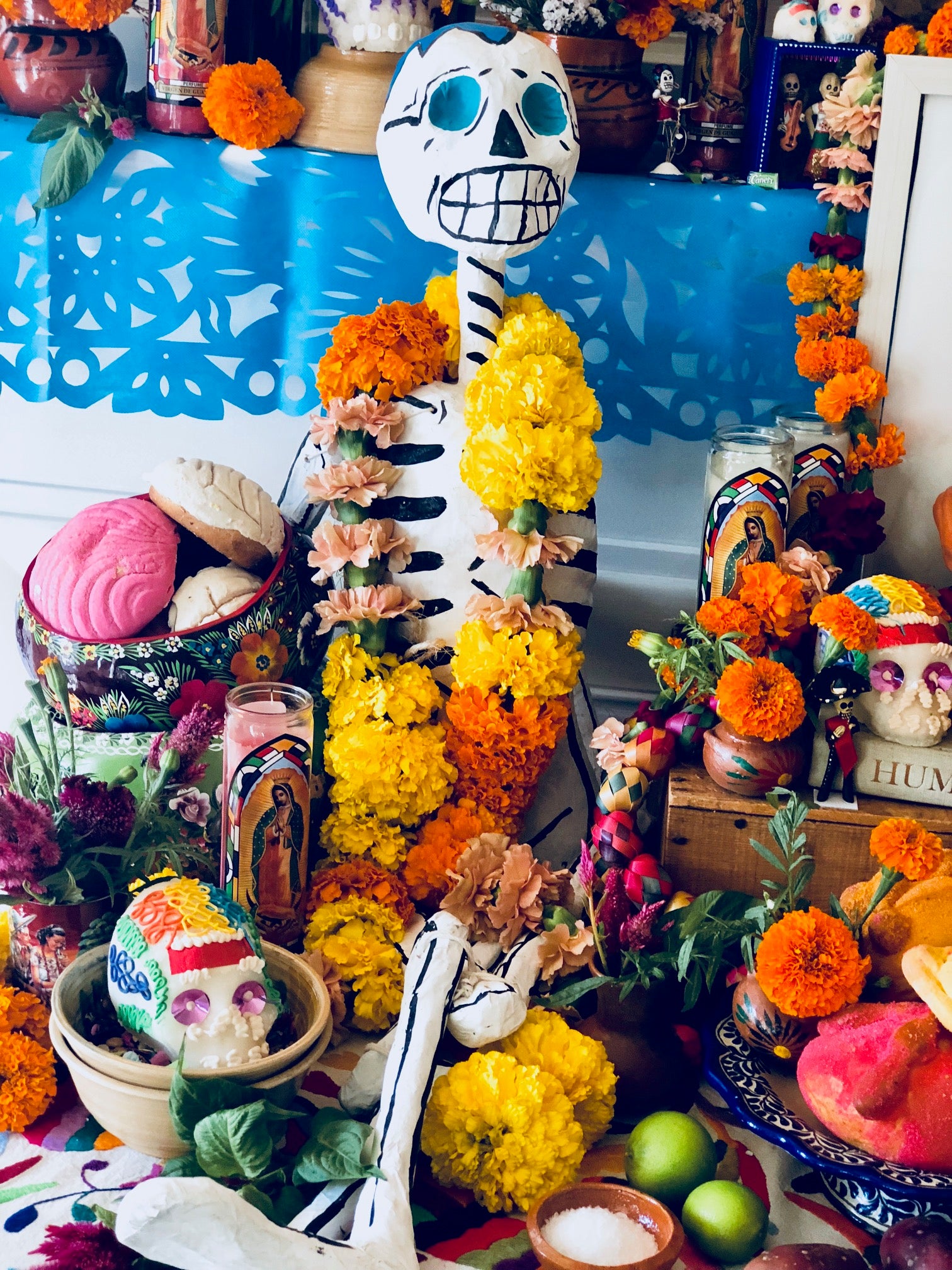In the vibrant and colorful image, a Day of the Dead display centers around a decorative skeleton figure, suggesting a celebration for the Dia de los Muertos. The skeleton, with a round white head, blue eyes, black nose, and an oval mouth drawn with teeth, wears a floral necklace made of orange, pink, and yellow flowers. It stands amongst a rich assortment of objects placed on a table. At the bottom right, there's a small brown bowl containing a white substance. Nearby, multiple green fruits, possibly limes or pears, are situated. A blue bowl with something pink inside, and two orange flowers are also visible.

To the left of the brown bowl, some yellow flower-like objects are positioned centrally. Adjacent to it, a long white object angles up and right across the frame, with a tan bowl containing a colorful, skull-like figure decorated with a red band across the forehead beside it. Behind this setup, a tall glass, and a bucket filled with cookies or muffins appear. Among the contents of the bucket are brown and pink items with white tops.

A leis of flowers drapes around a smaller skeleton, which features blue art at the top of its head, black lines down its neck, and horizontal lines on its body. The display is set against a blue background or covering, with a short white wall supporting an assortment of pots, a pot with an orange flower among other obscured items. The setup also includes bowls of sugar and a small white bowl of salt, emphasizing the festive and traditional elements of the Day of the Dead celebration. Various flowers, fruits, and decorative skulls contribute to the lively and meaningful atmosphere of the scene.